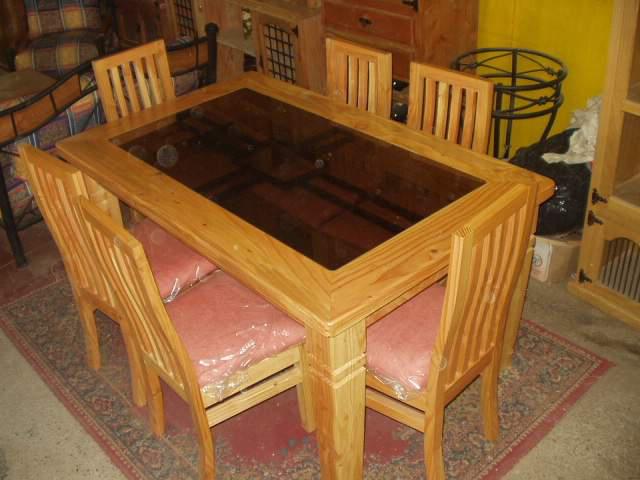This photograph captures a dining room set in an intimately lit home. Central to the image is a light-colored wooden table with a smoky, rectangular glass center supported by a metal structure. Around the table, there are six matching wooden chairs, all featuring salmon-colored cushions wrapped in protective plastic. The table and chairs rest on a faded, red Persian-style rug adorned with floral patterns and a pink border, beneath which a beige carpet with visible stains can be observed.

The room’s ambiance suggests a cozy but cluttered living space, with a mix of furniture and personal items. To the upper right of the frame, a piece of brown furniture with a black knob is positioned against the wall, which is either wood-paneled in an almost orange hue or painted yellow, depending on the lighting. Adjacent to this, a black metal plant stand stands empty. Additionally, a plaid living room chair and a couch, along with various bags and boxes, contribute to the room’s lived-in feel. The overall setting appears to be well-worn and slightly cluttered, hinting at a vibrant domestic life.